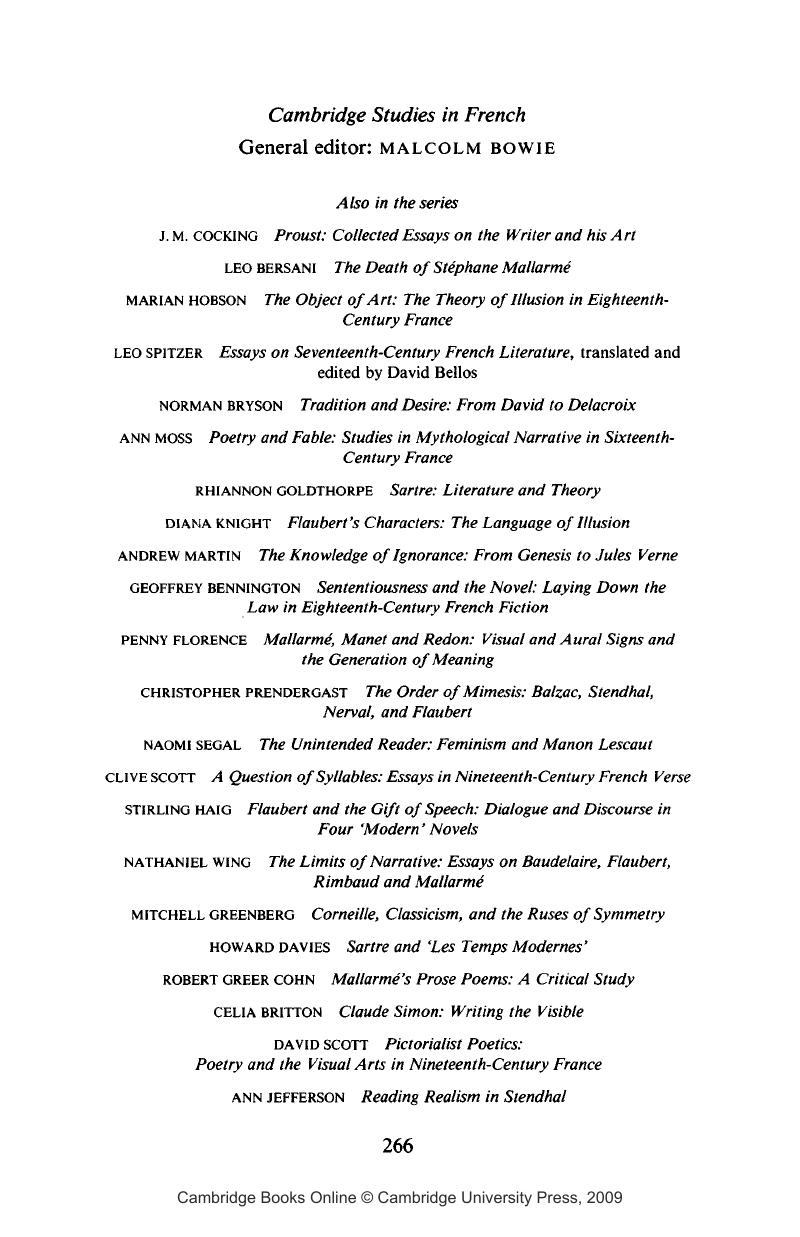The scanned image appears to be a white-background page from a book series catalog titled "Cambridge Studies in French," printed in solid black font. At the top, "Cambridge Studies in French" is italicized, followed by "General Editor Malcolm Bowie." The page lists various titles and authors in the series, starting with J. M. Cocking's *Proust: Collected Essays on the Writer and His Art*, Leo Bersani's *The Death of Stéphane Mallarmé*, and Marion Hobson's *The Object of Art: The Theory of Illusion in Eighteenth-Century France*. Other notable entries include Leo Spitzer's *Essays on Seventeenth-Century French Literature* (Translated and Edited by David Bellos), and Norman Bryson's *Tradition and Desire: From David to Delacroix*. Subsequent entries continue, featuring titles such as Anne Moss's *Poetry and Fable: Studies in Mythological Narrative in Sixteenth-Century France*, Geoffrey Bennington's *Sententiousness in the Novel: Laying Down the Law in Eighteenth-Century French Fiction*, and Daniel Wing's *The Limits of Narrative: Essays on Baudelaire, Flaubert, Rimbaud, and Mallarmé*. The page number 266 appears at the bottom, beneath which it states "Cambridge Books Online, Copyright Cambridge University Press 2009."